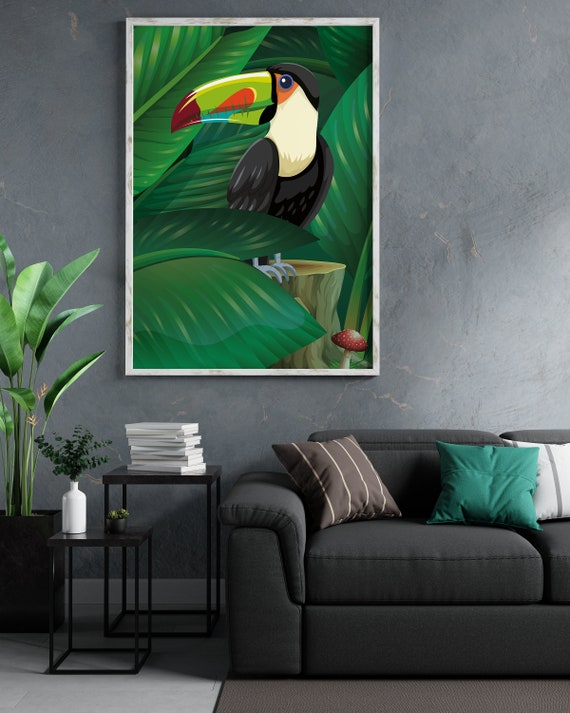The image depicts a stylish living room with a predominant gray theme. The focal point is a large, vibrant portrait of a toucan, featuring a colorful beak with shades of red, green, and orange, and surrounded by lush foliage that partially obscures the toucan's lower body. The background wall is painted gray, providing a neutral backdrop for the colorful artwork. Below the portrait, there is a navy blue couch partially visible, adorned with a variety of pillows: a striped green, brown, and white pillow; a white pillow; and a turquoise pillow. 

Adjacent to the couch is a small black end table holding a potted plant and a tiny object. A larger black planter containing a tall, striking plant stands beside the couch. In front of the couch, there's a coffee table with several white books stacked on it, though their titles are not discernible. The floor features a two-toned gray and brown rug that complements the overall color scheme. The room exudes a cool, laid-back vibe, accentuated by the cohesive interplay of vibrant art and minimalist decor.